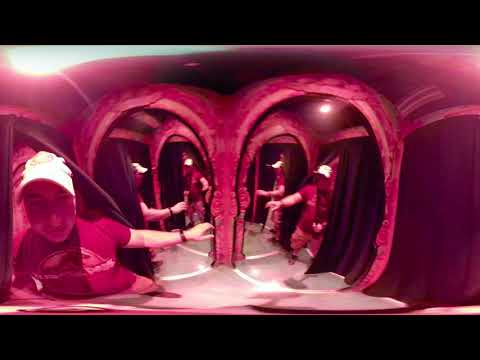The image is set in a hall of mirrors, likely an amusement park attraction, immersed in a vivid pinkish-red hue. The man in the scene, who appears multiple times due to the reflective surfaces, is wearing a white baseball hat, a gray (appearing red due to the tint) Jurassic Park t-shirt with cargo shorts, and a black bracelet on his outstretched arm. His image is reflected from various angles in at least five different places, creating a mesmerizing, distorted multiplicity. The central part of the photograph is dominated by two large mirrors with curved tops, bordered by straight sides, amplifying the visual echo. The intense red tint and reflections give the scene a twisted, almost surreal 360-degree flattened effect. To the right side of the mirror, a dark burgundy curtained entrance can be detected, while a bright white light illuminates the top left part of the image, enhancing the fantastical aspect of the visual experience.